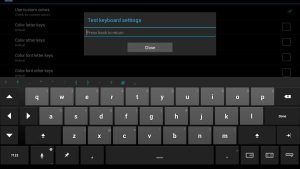The image depicts a device interface, likely a smartphone or tablet, oriented sideways. Dominating the screen is a virtual QWERTY keyboard featuring three rows of gray keys. The keys are primarily light gray with some accentuated by darker gray edging. Notable keys such as the backspace button are situated on the right, while arrow keys can be seen on the left. Towards the bottom, a space key and a microphone icon are clearly visible. Above the keyboard is a prominently displayed message in blue text that reads “Keyboard settings.” There is also an input field intended for user text entry, accompanied by a gray button with the word “Close” written in white. The background behind the keyboard is slightly darkened, with faint white headlines faintly visible on the left side, though the low resolution of the image makes the text difficult to discern. Overall, the focus is largely on the keyboard interface against the dimmed backdrop.